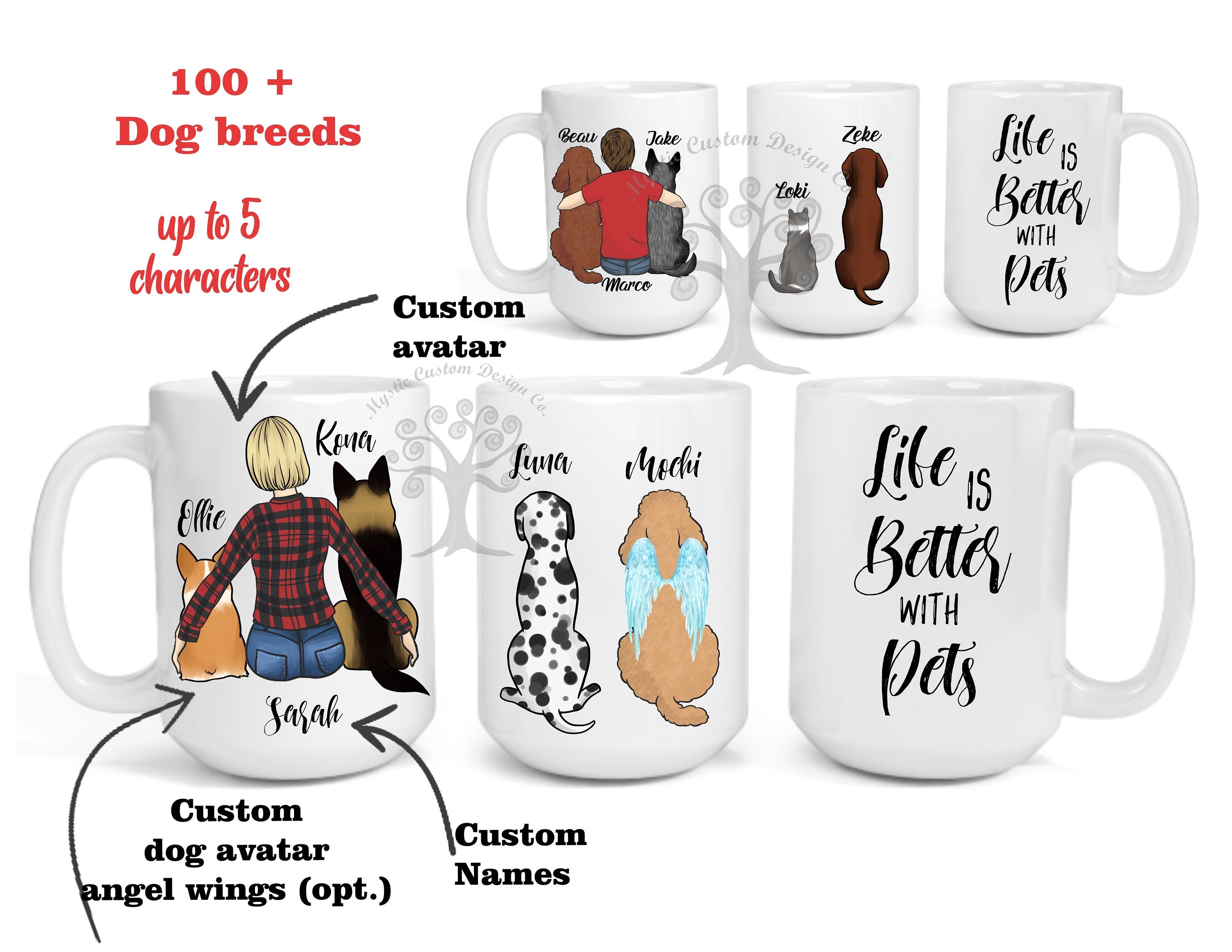The image is a vibrant, full-color collage composed of six different photos of white coffee mugs, arranged three on top and three on the bottom, set against a plain computer screen background. In the upper left-hand corner, striking red text reads "100+ dog breeds, up to five characters." Each mug features printed text and images. 

Starting from the left, the first mug displays Boo and Jake with a person named Marco holding the dogs. The second mug depicts a cat named Loki and a dog named Zeke. The third and fifth mugs, positioned on the right and the bottom row, respectively, both proclaim "life is better with pets" in white text. The fourth mug shows a woman named Sarah holding two dogs, Ellie and Connor. The sixth mug features two dogs named Luna and Muddy. Beneath some of the images are arrows pointing to additional text: "custom dog avatar angel wings optional" and "custom names."

Some names also appear in smaller text, including Ellie, Josiah, and Karen. There is also a visual element of angel wings on one of the dogs, suggesting it might be a memorial. The overall presentation is of personalized mugs featuring both pets and their owners, emphasizing the theme of remembrance and the joy pets bring to life.